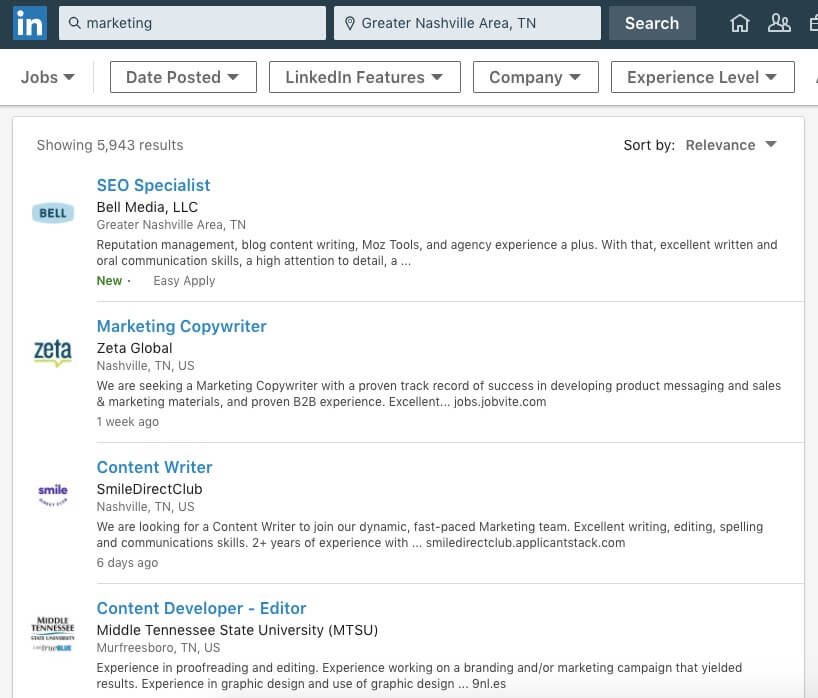The image depicts a search results page from Indeed, focusing on job listings related to marketing in the Greater Nashville area, Tennessee. At the top left corner of the page, the Indeed logo is prominently displayed. Adjacent to the logo, two search bars can be seen: the first one has "marketing" entered as the keyword, and the second one specifies "Greater Nashville Area, Tennessee" as the location.

Below the search bars, several filter options are visible, including "Date Posted," "LinkedIn Features," "Company," and "Experience Level," with selections made in each. The results display a total of 5,943 job listings, sorted by relevance.

The top listing is for an "SEO Specialist" at Bell Media, LLC in the Greater Nashville Area, Tennessee. The job description highlights requirements such as reputation management, blog content writing, familiarity with Moz tools, and agency experience as advantageous. It also emphasizes the need for strong written and oral communication skills and a high attention to detail, among other qualifications.

Following this, the second search result is for a "Marketing Copywriter" at Zeta Global, based in Nashville, Tennessee, USA. The job description mentions that the company is seeking a marketing copywriter, elaborating on the role's requirements.

The third search result features a position for a "Content Writer" at Smile Direct Club, located in Nashville, Tennessee, USA. The company is looking for a content writer to join their dynamic, fast-paced marketing team, requiring excellent writing, editing, spelling, and communication skills.

The fourth search result is for a "Content Developer/Editor" at Middle Tennessee State University in Murfreesboro, Tennessee, USA. This role involves experience in proofreading and editing, among other responsibilities.